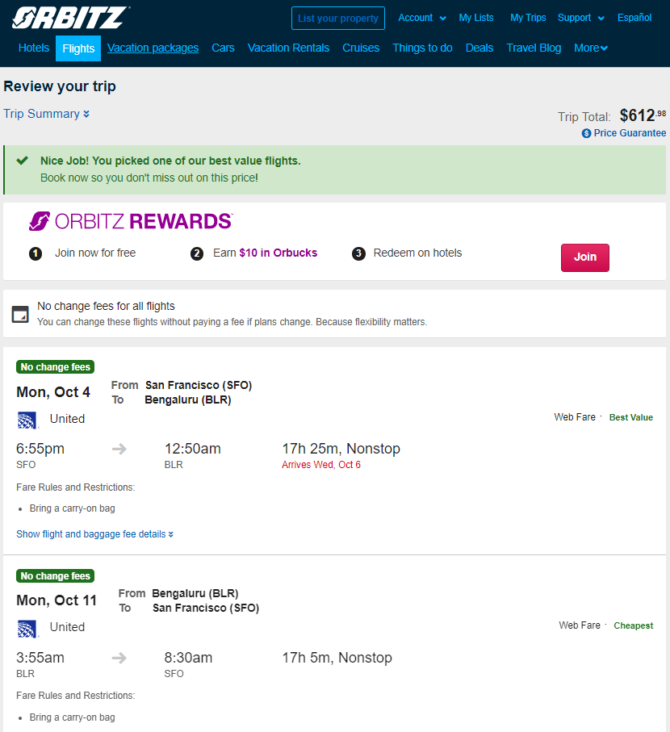This screenshot from the Orbitz website features a navy-blue header area with the Orbitz logo prominently displayed in white. The header also contains a user-friendly navigation bar with teal-colored text, offering quick links to various sections such as Hotels, Flights, Vacation Packages, Cars, Vacation Rentals, Cruises, Things to Do, Deals, Travel Blog, and More. Toward the center-top of the page, a teal-bordered button invites users to "List Your Property," while adjacent options include "Account" with a drop-down menu, "My List," "My Trips," "Support," and an option to switch the language to "Español."

As you scroll down, there is a section dedicated to reviewing your trip, featuring a detailed trip summary. Further down, the page promotes the Orbitz Rewards program, encouraging visitors to "Join Now for Free" and earn $10 in Orbucks, which can be redeemed on hotels. Below this, it provides a specific itinerary example, showing a travel period starting on October 4th and returning on Monday, October 11th.